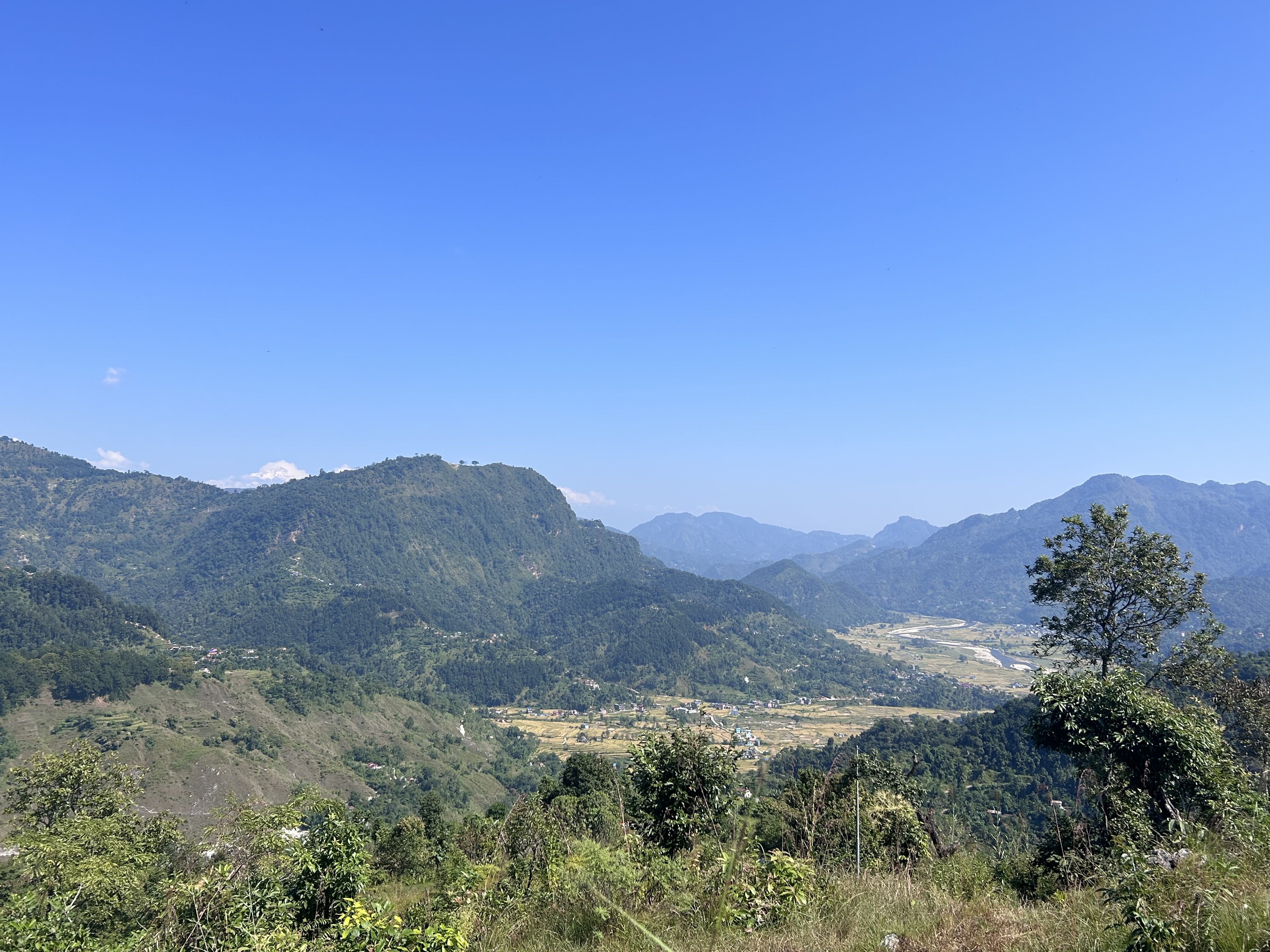The photograph depicts a scenic landscape featuring a significant mountain range and a lush valley. The mountains, covered in dense, green trees, stretch across the background with some exhibiting a bluish-gray hue, especially towards the horizon. The largest mountain stands out with a sheer cliff face, while another mountain slopes gently into the valley below. The sky above is a gradient of light blue, transitioning from a deeper blue at the top to a lighter shade near the horizon, dotted with white clouds. 

In the foreground, we observe tall green grass and bushes, indicating the vantage point is from atop a hill. Green leaves and some colorful flowers partially frame the image. The valley floor is intricately detailed, with a series of brick houses scattered throughout, hinting at a rural community. Dirt roads weave through the valley, possibly indicating farmland or small settlements. A road meanders along the lower hillside, where a cluster of houses can also be seen. The presence of these man-made structures, although somewhat distant and hard to discern, adds a layer of depth and context to the expansive natural beauty captured in the photograph.